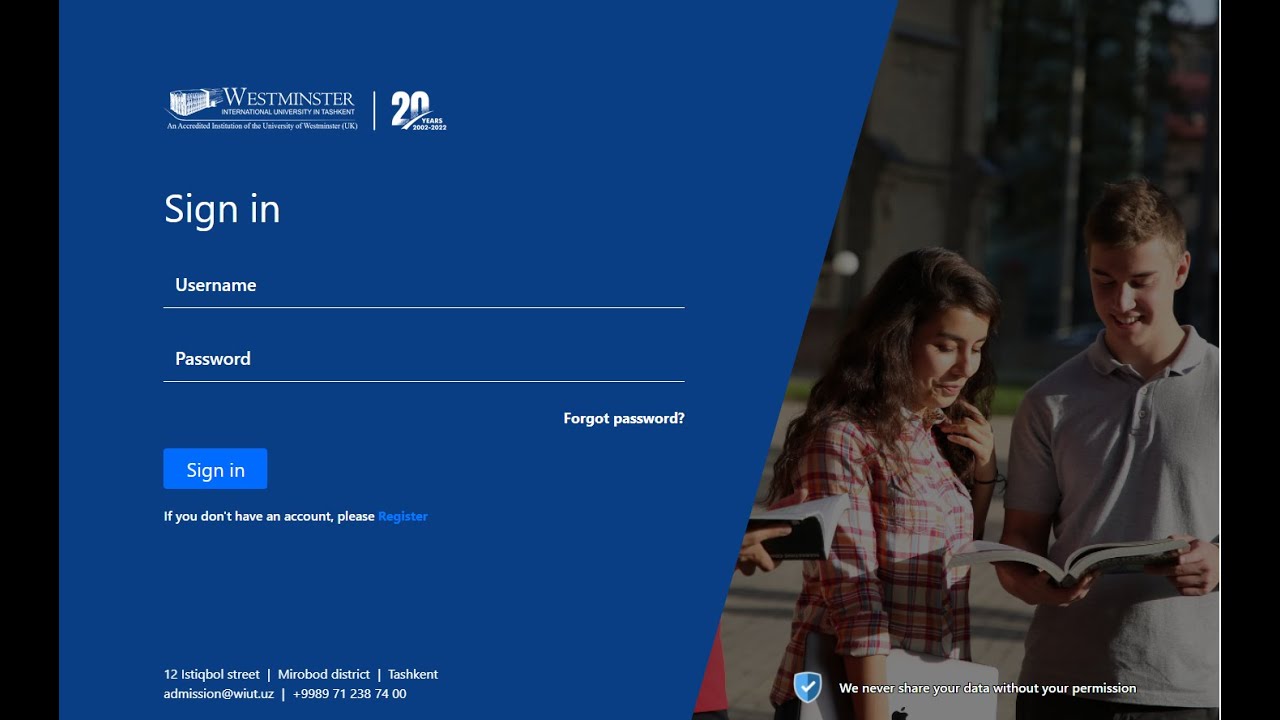In this detailed screenshot, we observe a vibrant image framed with black borders on the right and left sides. The main focus of the image is a young couple situated on the right side— the female is on the left and the male is on the right. Both appear to be smiling and engagingly looking down at a textbook held by the male. Overlaying the bottom part of this scene is white text stating, "We never share your data without your permission."

On the left side of the screenshot, set against a solid blue background, there are several elements. In the upper left corner, it reads, "Westminster International University in Tashkent," with a white illustration of a building to the left of the text. Adjacent to this is a commemorative text, "20 years 2002 through 2022," celebrating the university's anniversary. 

Below this, in bold white print, there is a prompt to "Sign In" followed by two input lines labeled "Username" and "Password." Near the lower right part of the password input line, there is a small white text link that reads, "Forgot Password." Beneath these fields, aligned to the left, is a blue action button labeled "Sign In." Just below this button, another message in white text invites new users with the line, "If you don't have an account please register."